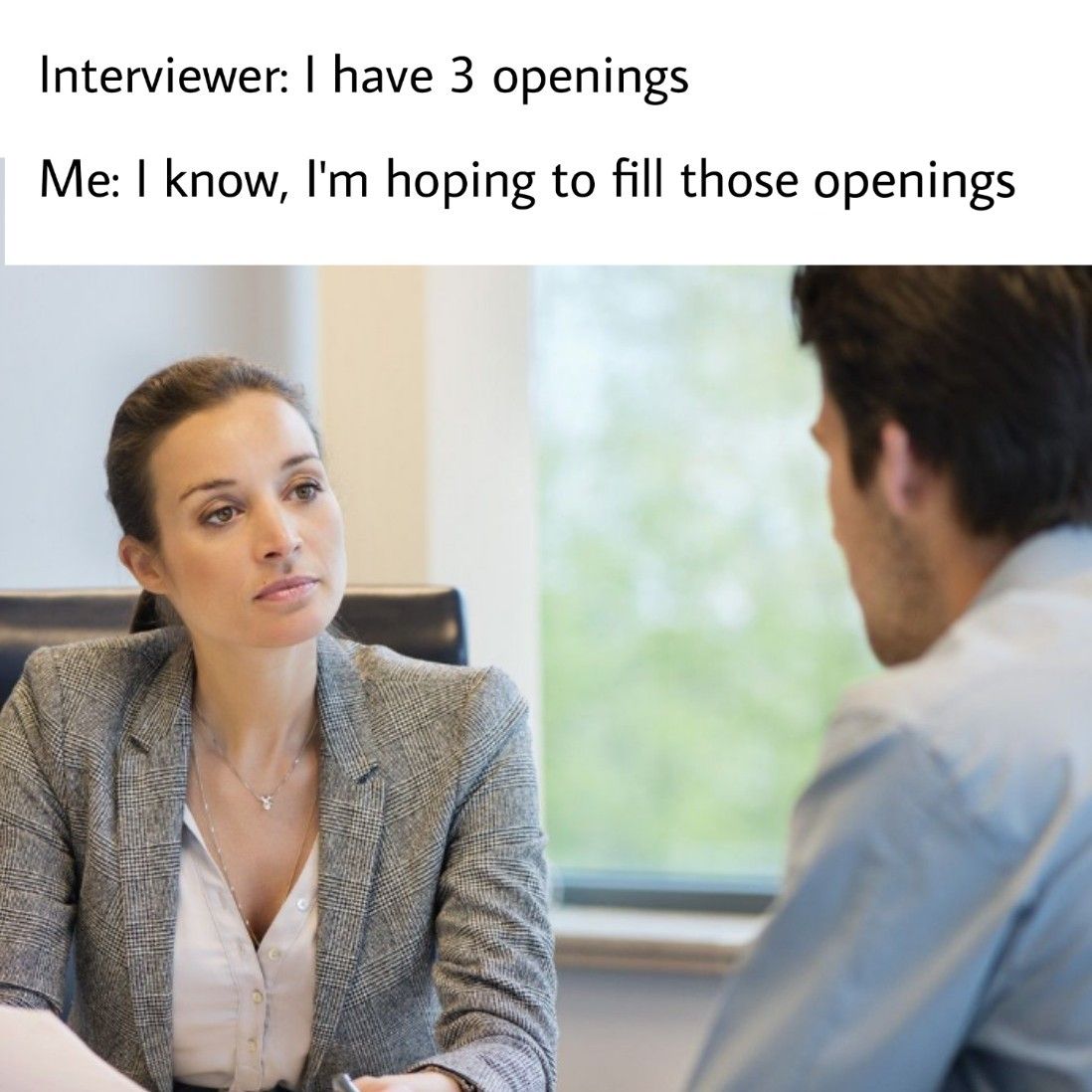This photo features an office setting captured during an interview. Dominating the scene is a woman who appears to be the interviewer, seated in a high-backed executive chair. She wears a white blouse beneath a brown plaid-patterned jacket, accessorized with a necklace. Her brown hair is neatly pulled back, and she has a serious expression, enhanced by her subtle makeup. To her left and partially blurred out is a man, likely the interviewee. He sports short brown hair, a scruffy beard, and a long-sleeved light blue shirt. The background showcases a large window on the right, slightly out of focus, contributing to the professional ambiance. At the top of the image, black text on a white background reads, "interviewer: I have three openings." Below that, it says, "me: I know, I'm hoping to fill those openings," indicating a playfully suggestive joke intended for online sharing.